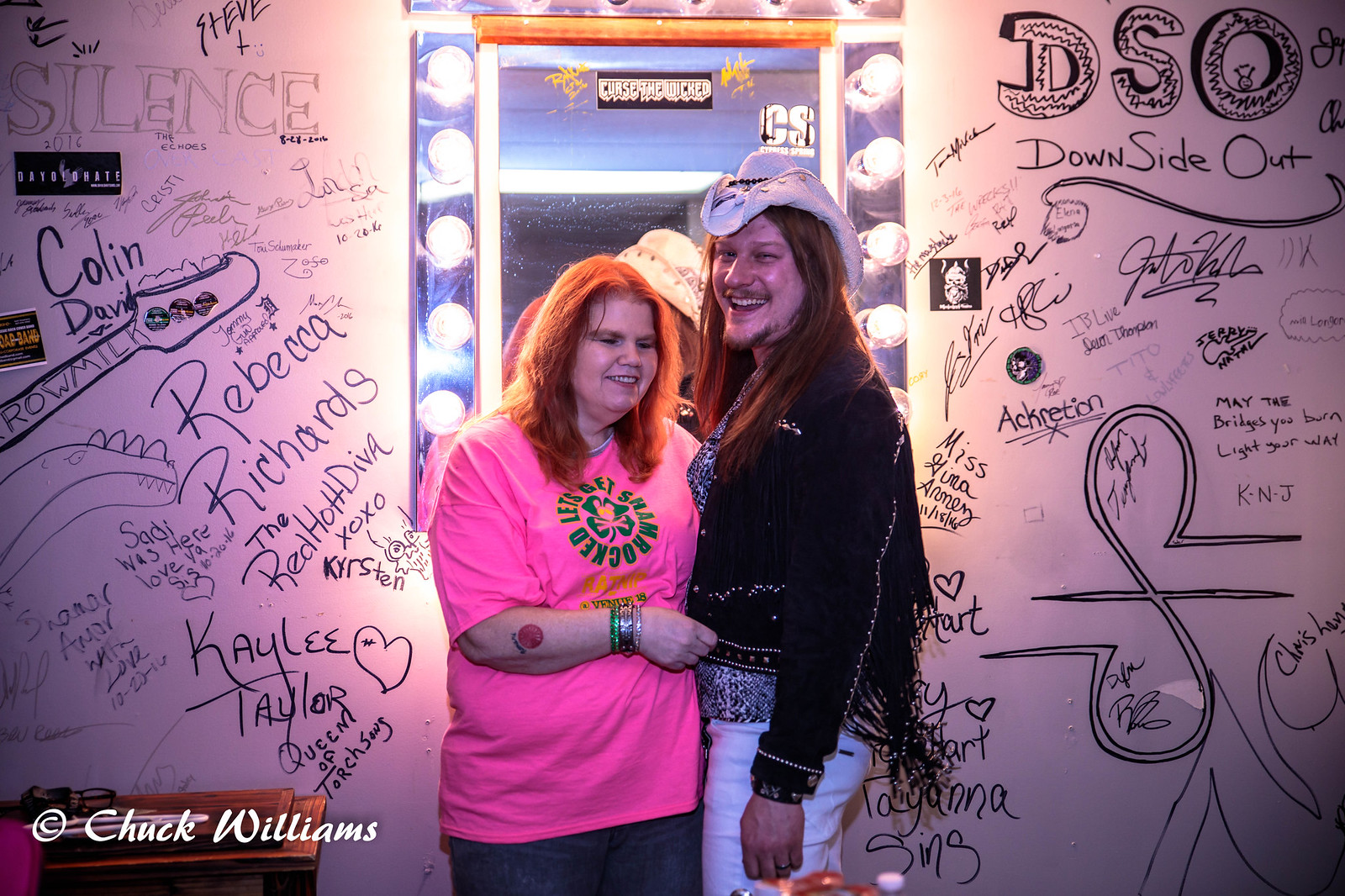This photograph by Chuck Williams, as indicated by the italicized copyright watermark in the bottom left corner, captures a man and a woman standing in front of a mirror adorned with large, round spotlight bulbs reminiscent of a theater dressing room. The white wall behind them is covered in various Sharpie marker signatures and messages, adding a personal touch from fans or visitors with names like Rebecca Richards, the Red Hot Diva, Kaylee Taylor, Queen of Torch Sins, Sadie Was Here, Colin David, Steve, DSO, and Downside Out. The woman stands to the left, wearing a pink t-shirt with green lettering that reads "Let's Get Shamrocked," blue jeans, and a mix of silver and green bracelets. Her ginger hair cascades to her shoulders, complementing the tattoo on her right forearm. To her right, but on the left side of the photo, the man dons a white cowboy hat and a black fringed jacket over a patterned black and white t-shirt. His long hair drapes down just above his chest, and he matches the look with white pants and a bracelet on his left wrist. Both are smiling, possibly at a meet-and-greet event, with their cheerful demeanor reflected in the mirror's light.